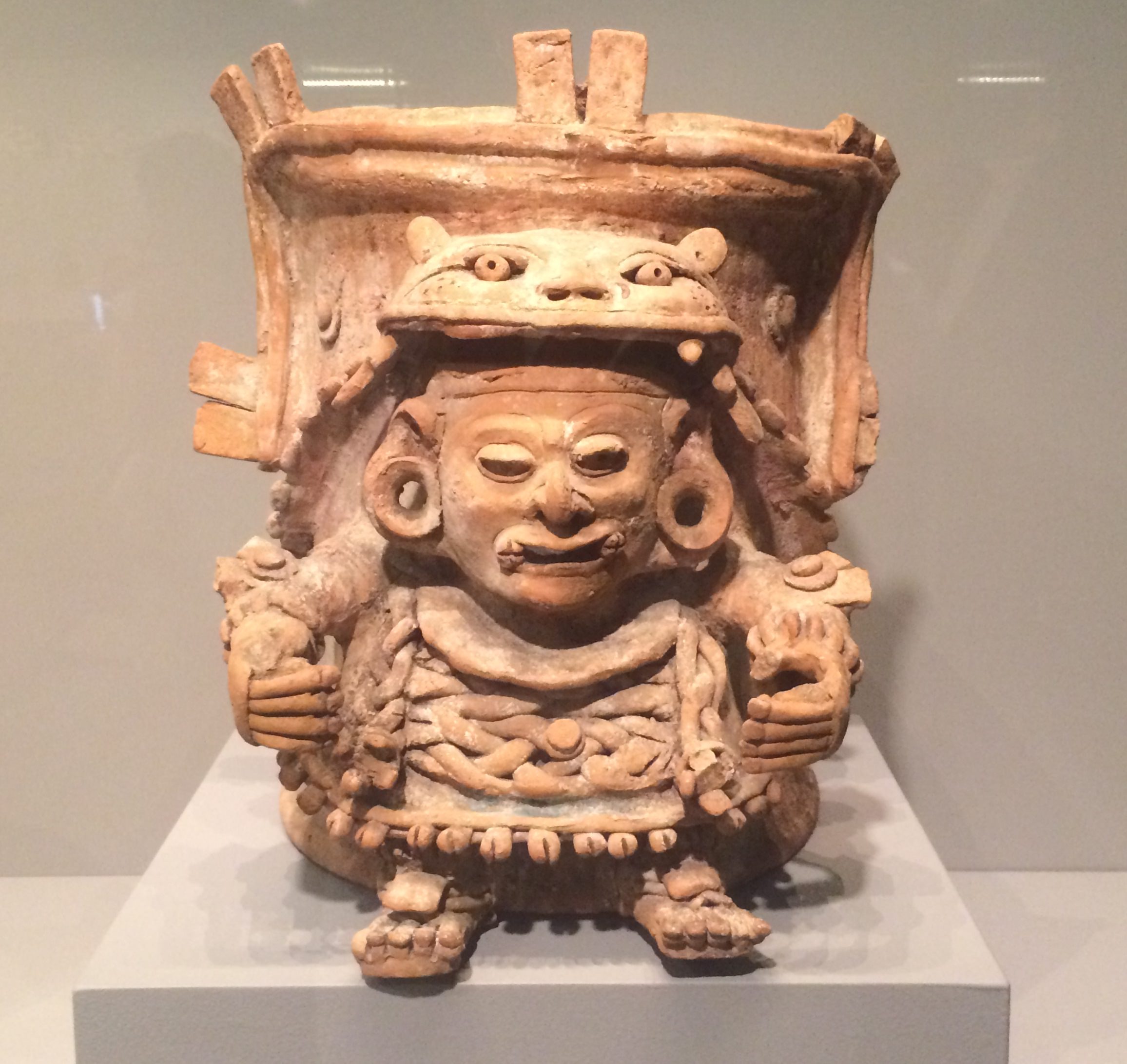This photograph captures a detailed terracotta-colored ceramic statue that appears to be an ancient artifact, potentially from the Aztec era. The central figure of the sculpture resembles a squat, mythological creature with distinct human and animal features. It has a short torso adorned with braided designs, flat feet, and hands, and large holes in its earlobes, presumably for earrings. Atop its head is the face of a large animal, possibly a cheetah or a hybrid of a frog and a bear, as if the creature is wearing the animal like a shroud. The statue, with its intricate details and ancient appearance, is positioned on a light gray platform, indicative of a museum display. Behind the sculpture is a wall exhibiting shades of tan, brown, and gray, complementing the statue's earthy tones. The entire setup emphasizes the antiquity and cultural significance of the piece, making it a captivating exhibit.